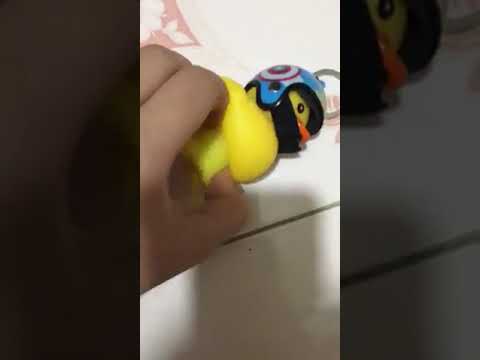This cryptic-style photograph features a person's left hand, showing only the thumb, index finger, and middle finger, holding a small rubber ducky. The yellow rubber ducky has an orange beak and wears a blue helmet adorned with a Captain America shield on the side. The ducky is lying on its side, angled diagonally to the upper right, and is placed on a white surface, possibly a table. The background includes a white sheet with some pink markings, and the upper left corner has additional pink and white elements, possibly seams resembling caulk in tile. The image is structured with a center panel in focus and two blurry side panels, framed by a relatively thick border on both sides. There's no text in the photo.